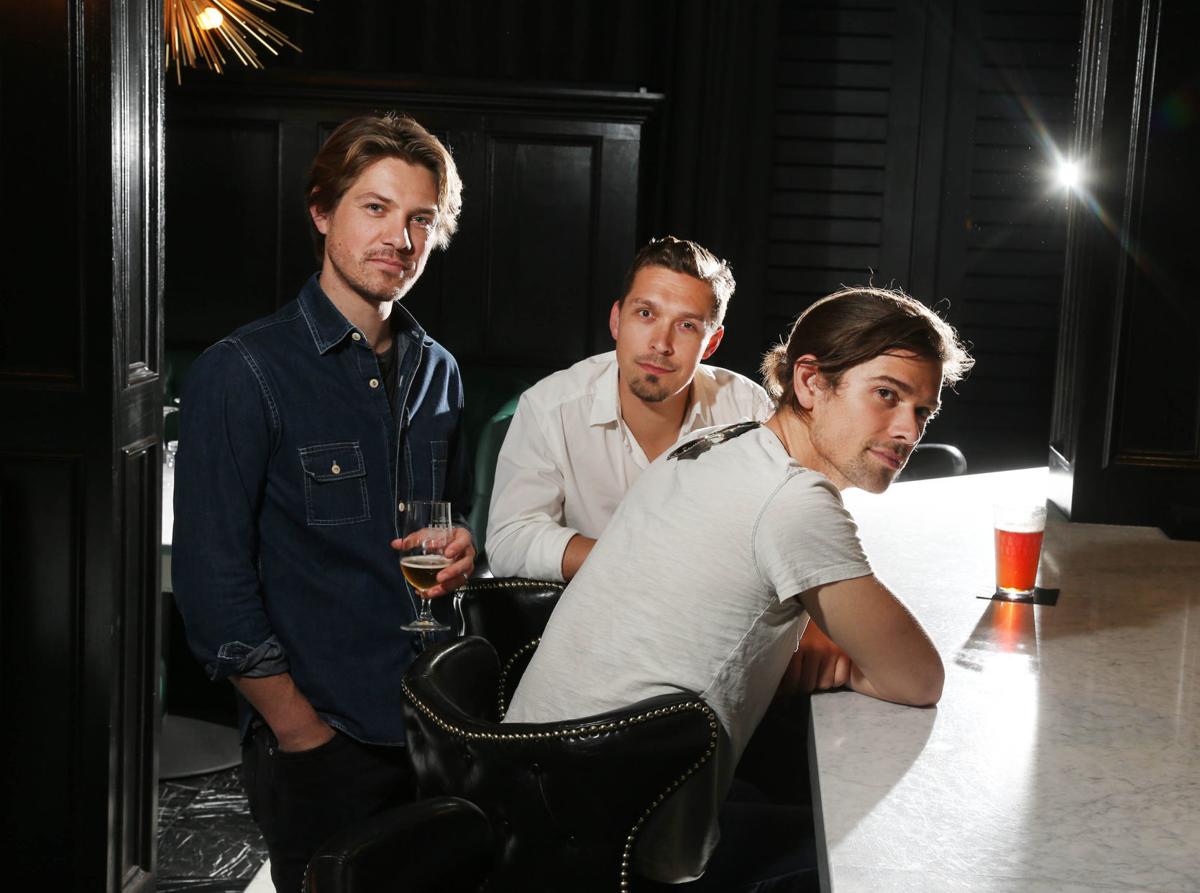The image depicts the grown-up members of the band Hanson sitting at a bar with a contemporary ambiance, featuring black walls, subtle lighting, and white countertops. The three brothers are positioned at high-top bar stools with black leather backs. The youngest brother on the left, dressed in a white shirt and with long hair tied back in a ponytail, gazes over his right shoulder towards the camera. The middle brother, wearing a blue denim shirt and sporting scruffy facial hair, is standing and holding a half-drunk glass of beer in his left hand. The oldest brother is seated furthest to the right, clad in a white button-down shirt, with short hair and a goatee, staring directly at the camera. The setting is accentuated by muted lighting, creating a cozy, intimate atmosphere.